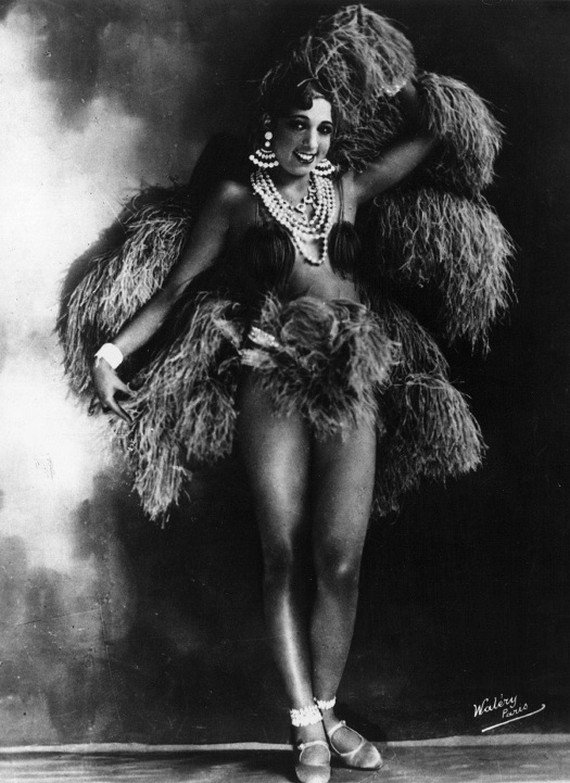The image depicts a striking black and white photograph of the iconic dancer Josephine Baker. She stands confidently in a poised stance, her left arm extended upward holding what appear to be pom-poms or elaborate feather arrangements, and her right arm pointing downward near her hip. Baker, a beautiful dark-skinned woman with short, wavy black hair, is adorned with an abundance of pearl jewelry, including long earrings, multiple necklaces, and a bracelet on her left wrist. Her attire is minimal, with her body mostly uncovered, save for strategically placed black circular coverings over her breasts and feathered pom-poms around her waist and hips. She wears white sandals or slipper-like shoes, and her legs are fully visible. Behind her, the background transitions from white and gray to a solid black on the right, creating a dramatic contrast. The photograph is signed at the bottom right, "Wallery Perisco," underscored with a line. The image showcases Baker's radiant smile and graceful pose, capturing the essence of her legendary career as a performer and showgirl.